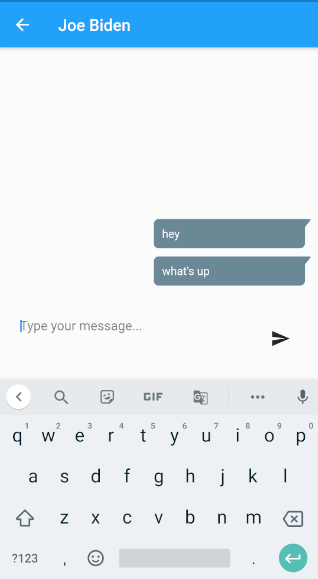This is a detailed description of a mobile device screenshot. At the top of the screen, there is a blue rectangular banner. On the left side of this banner, there is a left-facing arrow button indicating a back option. Within the blue rectangle, text identifies the recipient of the message as "Joe Biden."

Below the blue banner, there are two text message bubbles aligned to the right. The first bubble contains the message "Hey," and the second one below it reads "What's up?"

Underneath these text bubbles is a text input field with the placeholder text, "Type your message..." and a small icon suggesting where to press to send the message.

Below the text input field, the phone's keyboard is displayed. Above the keyboard, there are several function buttons, including a magnifying glass icon for search, a sticky note with a smiley face for adding emojis, a button labeled "GIF" for sending animated images, and the Google Translate logo indicating a translation feature. An ellipsis icon is present, signifying additional options.

Below these function buttons is the standard QWERTY keyboard. Each key from Q to P has a corresponding number from 1 to 0, continuing the convention of standard keyboard layouts.